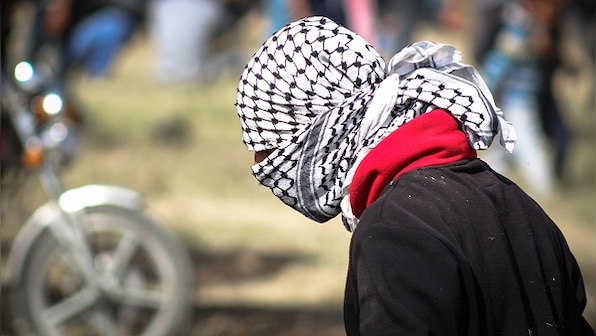In this vibrant daytime photograph taken outdoors, the focal point is a side-profile portrait of a man, strikingly dressed in traditional Middle Eastern attire. His head and most of his face are wrapped in a black and white checkered keffiyeh, iconic in design and typically associated with Palestinian culture. The scarf is meticulously tied at the back of his head, leaving only a narrow slit open for his eyes. Below the keffiyeh, he wears a thick red scarf around his neck and a dark, possibly black, jacket that adds to his layered clothing ensemble.

The background, rendered in a soft blur to emphasize the subject, features the front wheel and headlight of a motorcycle, adding an element of rugged scenery to the setting. The ground beneath is a blend of beige-colored concrete and a darker road surface. Additionally, faint outlines of people, dressed in white, blue, and pink, can be seen strolling, hinting at a bustling cityscape. The sunlight bathes the entire scene, ensuring the man stands out prominently against the softer, indistinct backdrop. This moment, seemingly set in the Middle East, captures a rich tapestry of cultural and urban elements, unified in a single frame.